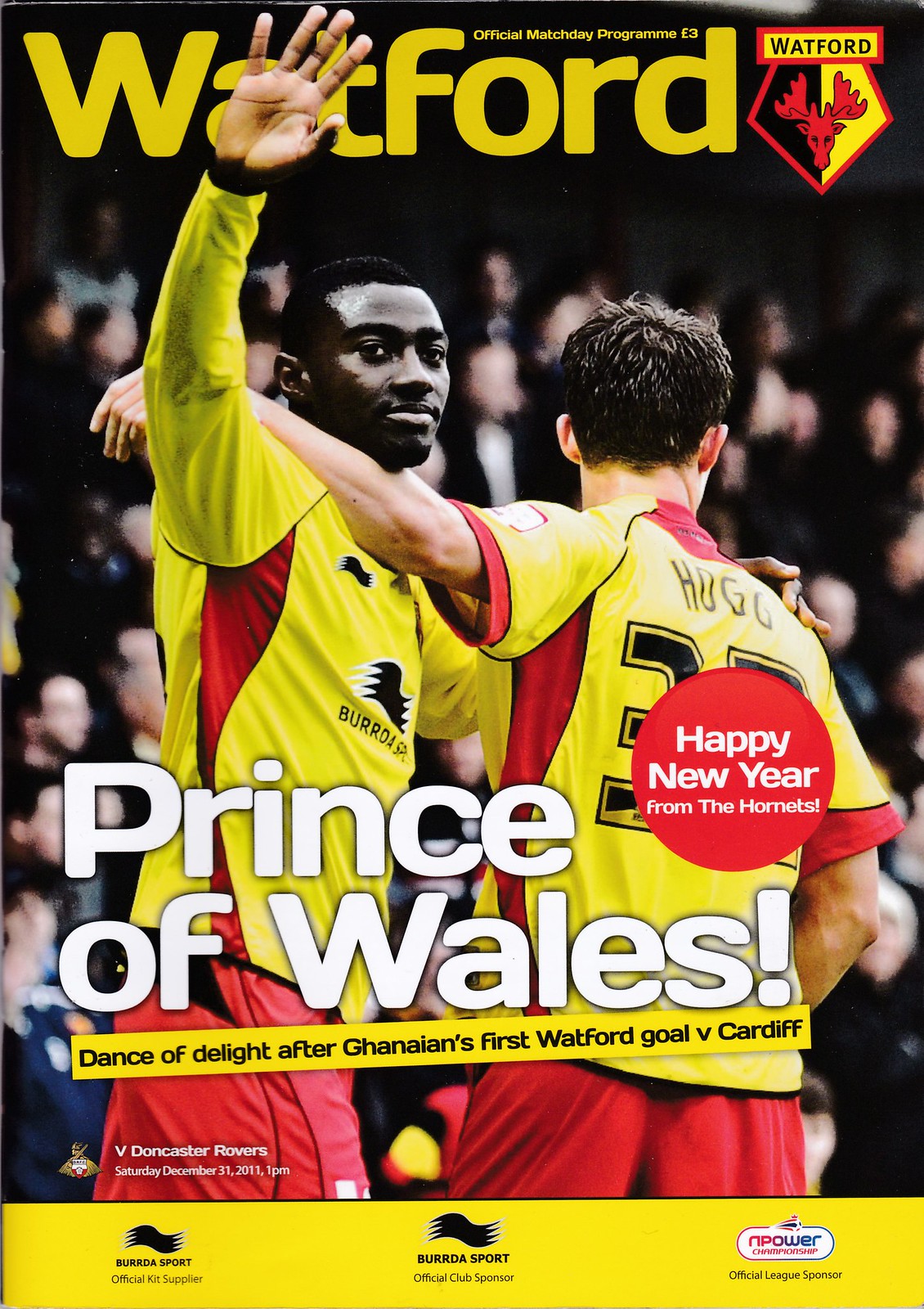The cover of the official match day program for a Watford FC soccer match is prominently displayed. At the very top, in yellow font, it reads "Watford," with smaller text above that stating "Official Match Day Program Three Pounds." The Watford emblem, depicting a red moose head with antlers against a yellow and black background, is also featured prominently. Below the title, in large white font, it reads "Prince of Wales," highlighting a celebratory article titled "Dance of Delight After Gannon's First Watford Goal Versus Cardiff." A red circle adds festive cheer with "Happy New Year from the Hornets." The main image shows two players in yellow jerseys with red and black accents and red shorts. One player, with "Hugo" on his jersey, faces away from the camera with his left hand on his teammate's shoulder. The other player, waving his right hand, faces the camera. The bottom of the program details the match against Doncaster Rovers on Saturday, December 31, 2011, at 1 p.m. Sponsors listed at the bottom include "Berta Sport" as the official kit supplier and "In Power Championship" as the official league sponsor. The background subtly features a blurred crowd, adding to the lively atmosphere of the cover.